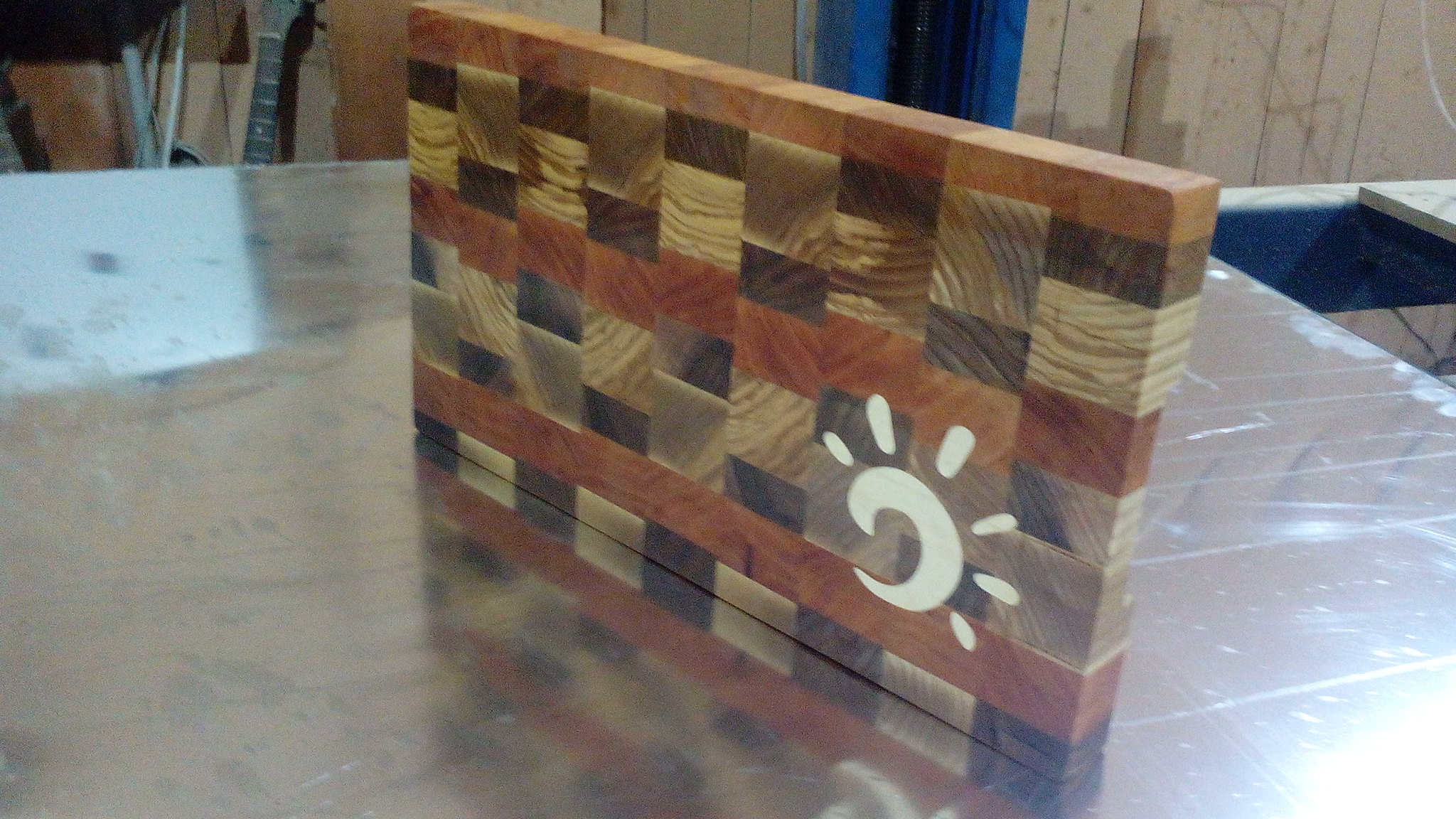The image displays a workshop table with a laminated wood top, partially reflective and showing signs of use with scratches and streaks. The backdrop is a paneled wood wall. On the upper left side of the image, guitar necks are visible, suggesting that the space might belong to a luthier. Centered on the table is a distinctive block, constructed from various squares of wood, resembling a checkerboard with its diverse pattern. This pattern features shades of light beige, almost black, reddish-brown, and chocolatey brown, with some stripes of red oak. Each wooden square or rectangle varies slightly in size, contributing to a unique mosaic effect. Towards the lower right of the image, an abstract logo is overlaid, featuring a curved, wave-like design with white blotches and a series of elongated ovals or lines emanating from it, reminiscent of a stylized sun.